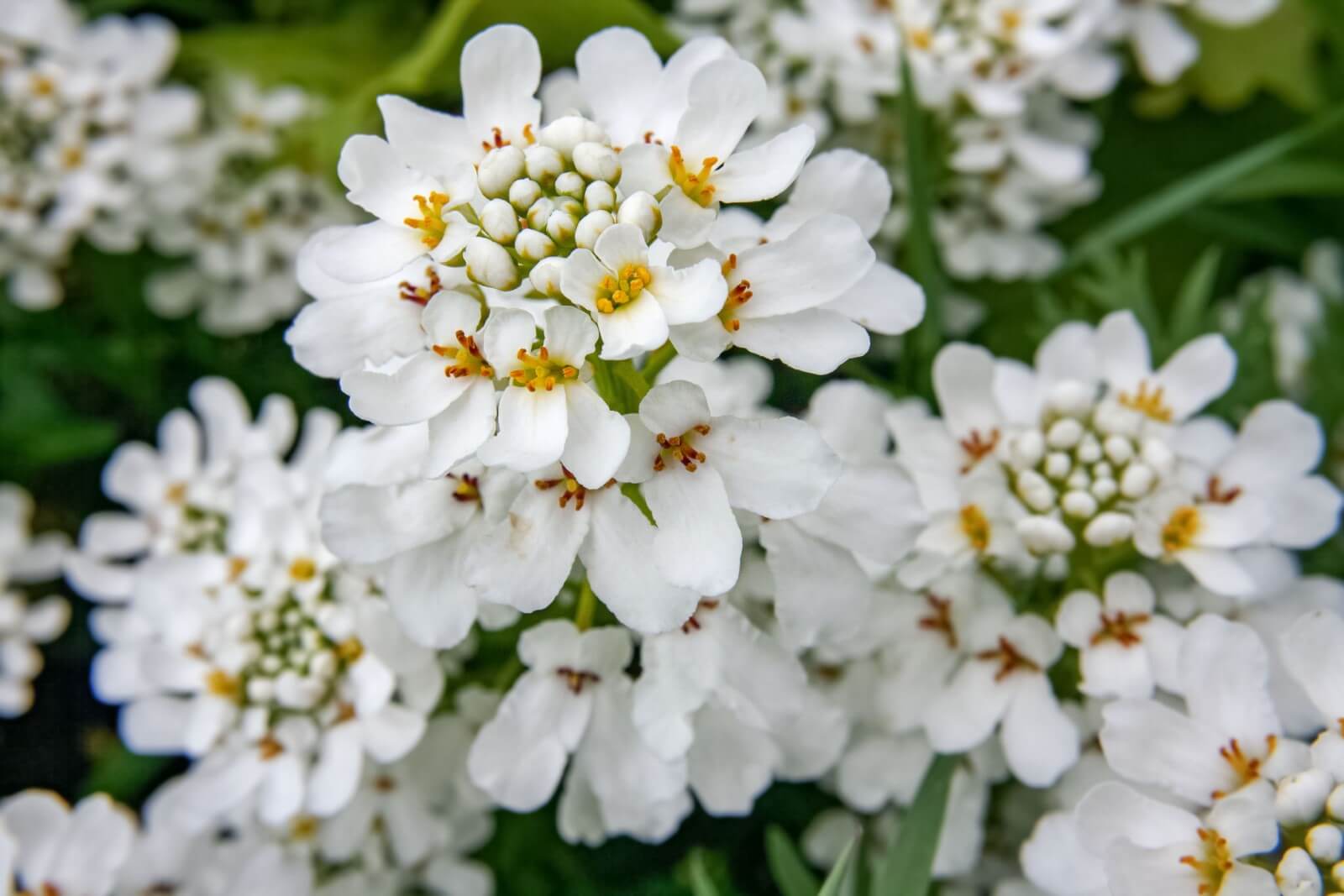This detailed image is a close-up photograph of white flowers with a focus on a central, prominent bloom that fills the forefront. The focal flower features about 20 white petals, with a composition further enriched by white and yellow spherical elements at its center, and some yellow-green and yellow-red hues adding to its intricate detail. This flower is showcased clearly, while the surrounding flowers, leaves, and stems, which are identical in type, gradually blur toward the background, creating a depth effect. The greenery of the stems and leaves, although present, is not the main focus and appears interspersed among the flowers. The background at both the top and bottom of the image is softly blurred, and the lighting throughout the picture is even, likely indicating a cloudy day with no sharp highlights. The overall color palette is composed of whites, varying greens, yellows, and subtle hints of red, providing a rich yet softly blurred backdrop to the standout white petals of the central flower.